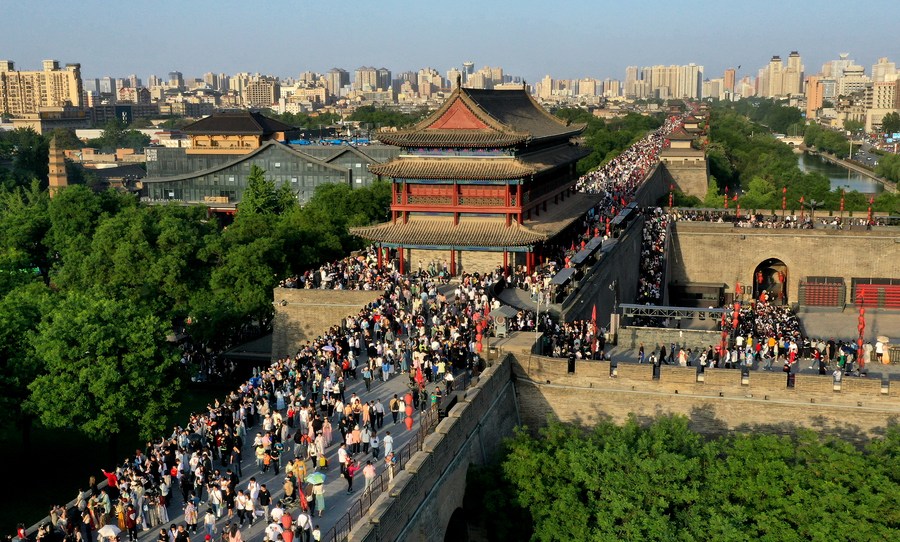This image is a detailed aerial photograph capturing what appears to be the Great Wall of China. In the foreground, the wall extends diagonally from the lower left corner, stretching off into the distance where it meets a vast city skyline. This cityscape is marked by numerous towering skyscrapers, some of which are taller than others, creating a bustling urban backdrop. 

Dominating the middle of the wall is a tall, traditionally Chinese building adorned in hues of red, brown, and black, standing prominently amidst the vast structure. The wall itself is crowded with what looks to be hundreds, if not thousands, of tiny, indistinguishable people, creating a continuous stream of activity along its length. 

On either side of the wall lies a verdant landscape, with bright green trees dotting the area, lending a stark contrast to the gray of the wall and the urban sprawl beyond. The photograph was taken on a clear, sunny day, evidenced by the blue sky devoid of clouds, which stretches across the top of the image. This harmonious blend of ancient architecture, natural greenery, and modern cityscape vividly captures the essence of this significant historical monument and its surroundings.